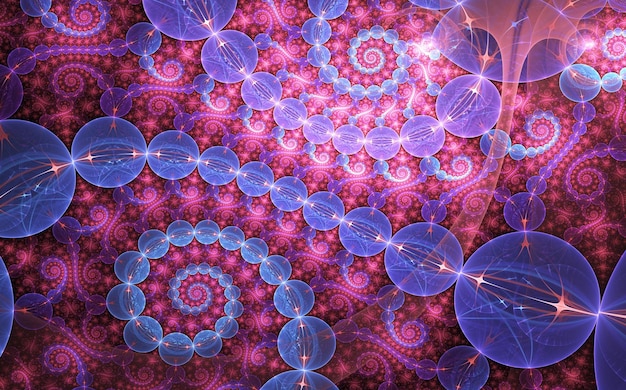The image presented is a detailed piece of psychedelic digital art with a rectangular format. The background features vivid pinks and light pinks, intertwined with patterns of gold and white that resemble paisley designs. Adding depth to the background are purple swirls that form spiral patterns, enhancing the overall psychedelic effect.

Dominating the foreground, there are multiple vibrant blue circular patterns that resemble beads or chains of beads. These circles form two primary spirals: one extends from the bottom right to the middle left, spiraling intricately on the lower left, while another is more concentrated in the top center, looping tightly within itself. These blue circles are illuminated from within by golden lights, resembling stars or glitters, giving them a radiant, almost fluorescent glow. This inner illumination is most prominent in the top center spiral, where the brightness reaches a whitish hue, further emphasizing the luminous quality of the art.

The combined elements of blue luminous circles, gold star-like lights, and harmoniously intertwined pink and purple patterns create a complex and mesmerizing visual experience, evoking the intricate structures of the brain or a deeply psychedelic realm.